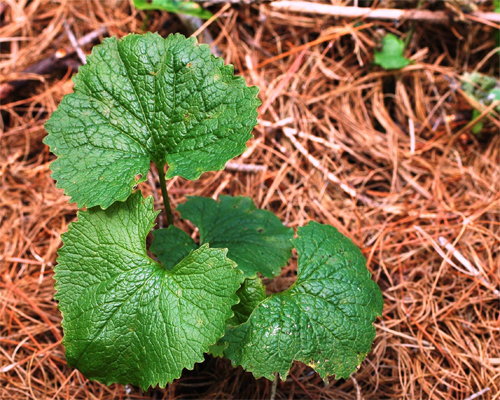This overhead close-up photograph captures a vibrant green sapling growing amidst a bed of dried, orange pine needles. The central focus is on the small plant with four semi-circular, jagged-edged leaves that radiate from a central swirl, displaying prominent veins. These leaves have a shiny texture and are a lighter green with deeper-colored veins, creating a striking contrast against the pine-needle-covered ground. Scattered across the foreground are small sticks and twigs, with additional, slightly blurred smaller saplings visible in the background. A few leaves on the plant have tiny holes, possibly from insect activity, adding a touch of natural imperfection to its otherwise lush appearance.